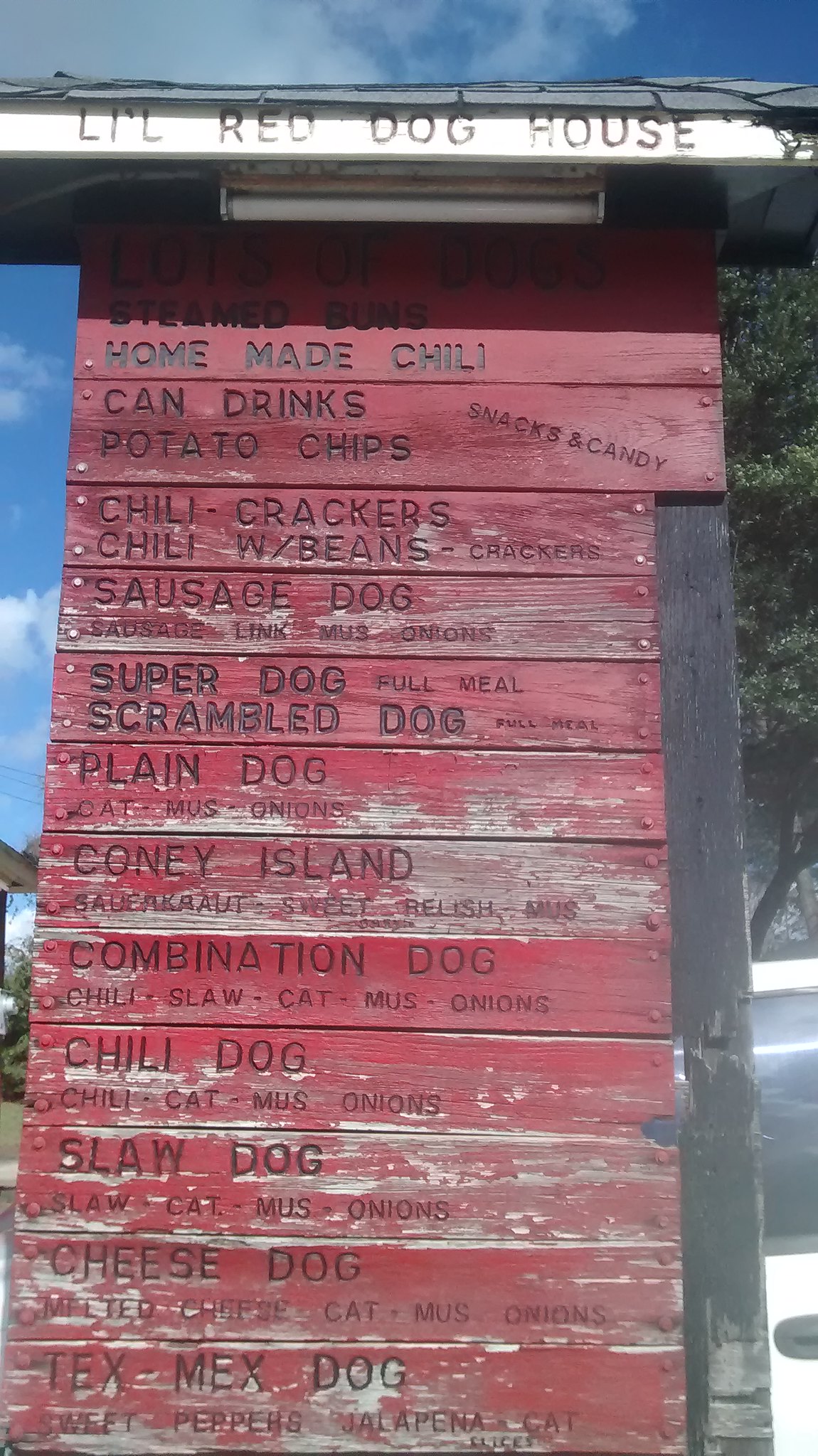The image showcases a rectangular photo of an outdoor menu sign for a food truck or restaurant. The tall wooden sign, constructed from wooden planks painted red with some white spots indicating worn-off paint, features black, engraved lettering that appears to be burned into the wood. The sign is topped with a white header reading "Little Red Dog House," underneath which there's an installed but unlit fluorescent light bulb.

The menu items listed on the sign include:
- Lots of Dogs
- Steamed Buns
- Homemade Chili
- Canned Drinks
- Potato Chips
- Snacks and Candy
- Chili Crackers
- Chili with Beans
- Crackers
- Sausage Dogs
- Sausage Link
- Mustard & Onions
- Super Dog
- Full Meal Scramble Dog
- Full Meal Plain Dog
- Coney Island
- Sauerkraut
- Sweet Relish
- Mustard
- Combination Dog
- Chili Slaw
- Chili Dog
- Slaw Dog
- Cheese Dog
- Melted Cheese
- Tex-Mex Dogs
- Sweet Peppers
- Jalapeños

Additionally, the sign mentions extra toppings and combinations such as "ketchup mustard onions" (abbreviated as Cat Muss Onions), appearing multiple times throughout the menu. The photograph is taken during daylight, and a white car can be seen in the background, enhancing the outdoor setting.